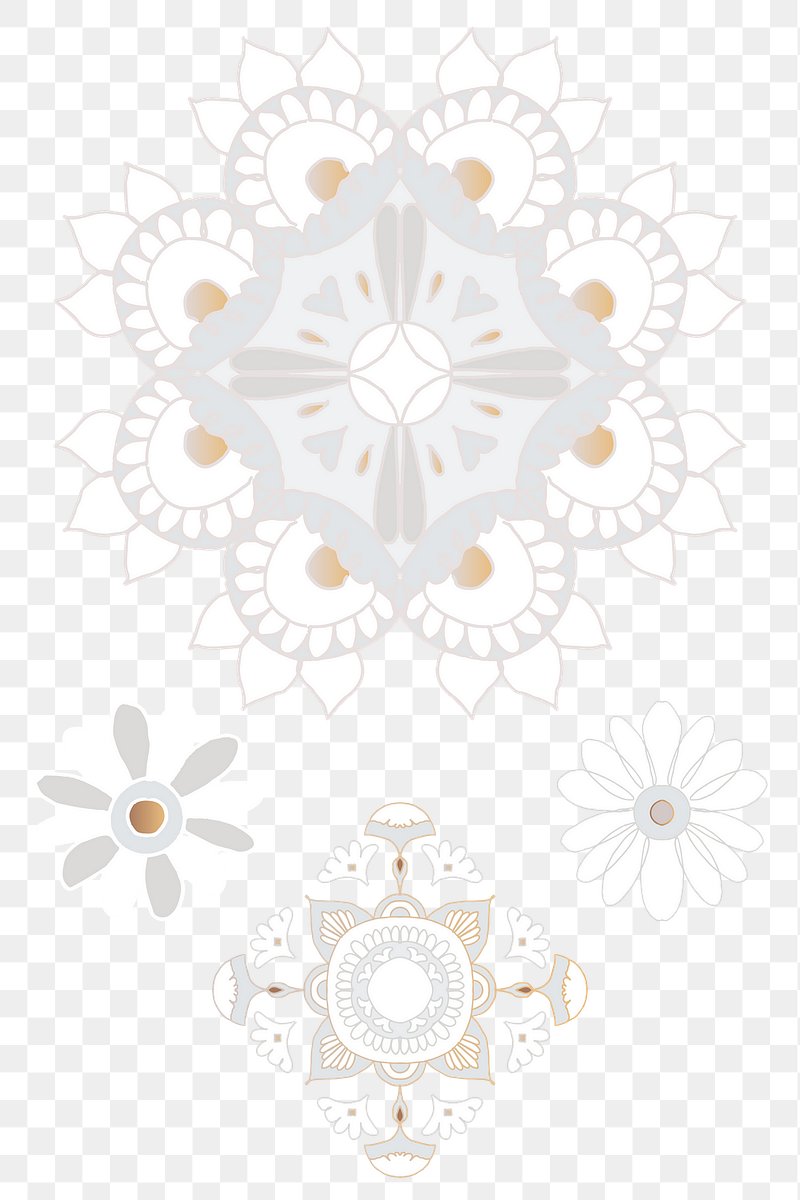The image is a detailed piece of computer-generated art featuring a white and gray checkerboard background with 44 rows of squares. Dominating the top half of the rectangular image is a large floral pattern, occupying 25 of the 44 rows. This intricate design has a white center with triangular tips, surrounded by dark grey flowers and interspersed with white circles that have yellowish centers. Below this central decoration are three smaller symbols: on the right, a white flower with many petals; on the left, a grey flower with six petals; and at the bottom, a square shape made of flower edges. The overall design is faint and grey, with subtle hints of orange, creating an abstract, kaleidoscope-like effect with repetitive floral and geometric motifs, including hearts, circles, and leaf-like shapes.